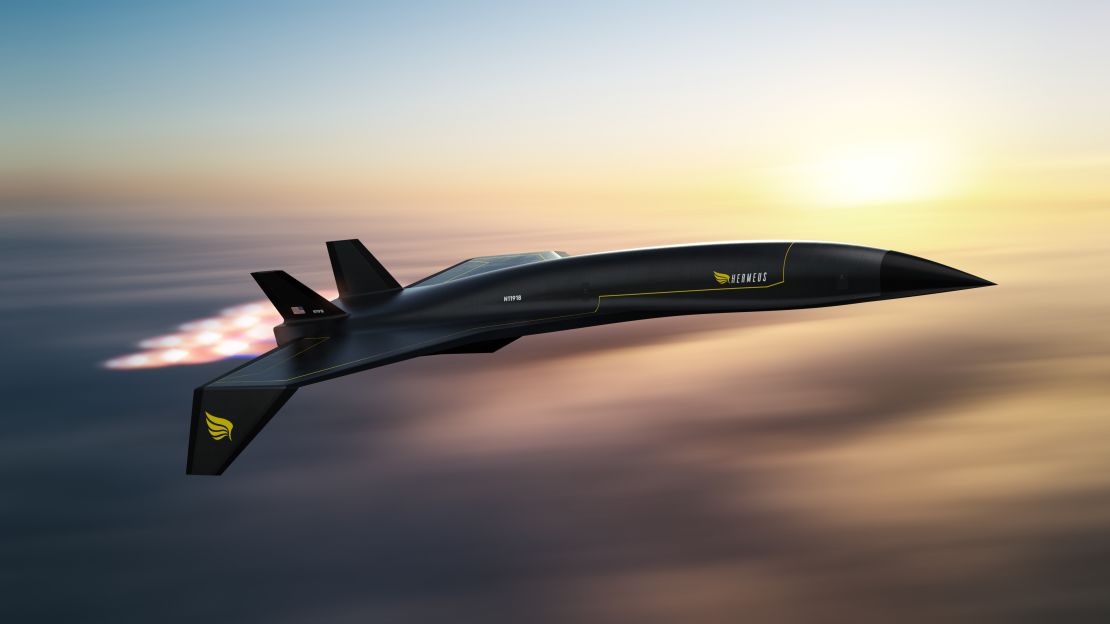The image is a concept piece showcasing a sleek, black aircraft, possibly a military jet or a supersonic passenger liner, flying at extremely high speeds. The plane, marked by undecipherable white text and adorned with a yellow wing logo featuring four sections and a possible gold triangular logo or flower on one of its tail fins, stands out sharply against a blurred sky backdrop. The sky gradient transitions from a light blue at the top to dark gray and light yellow toward the horizon, suggesting a sunrise or sunset. The aircraft flies horizontally with a prominent white and red engine trail, indicating supersonic speeds, and features tiny wings towards the rear with downturned tips. The tail number, although in white, is not clearly visible. The overall scene captures the dynamic energy and futuristic design of the aircraft against a dramatic, colorful sky.